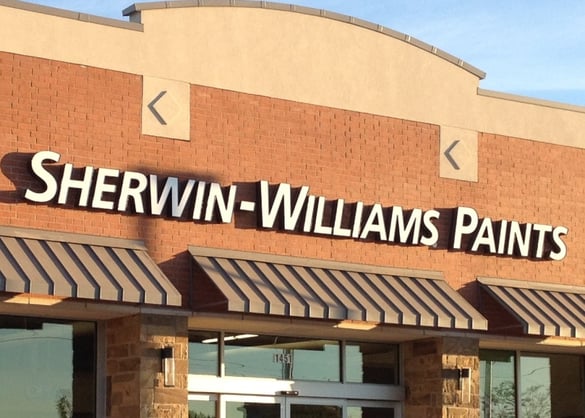The image captures a Sherwin-Williams paint store, characterized by its distinctive architecture. The building features an orange-red brick facade with a smooth upper section made of a pinkish stone material that arches gracefully towards the center. The store name, prominently displayed in large white capital letters, casts a noticeable shadow on the building due to the sunlight. Below the sign, three gray awnings equipped with fluorescent lights extend over the entrance. The lower section of the building showcases tall windows and the address number "1451" in black and white square letters positioned above the door. Flanking the entrance are two light fixtures, clear at the bottom and dark at the top. The entrance itself consists of an automatic door that seamlessly opens for visitors.